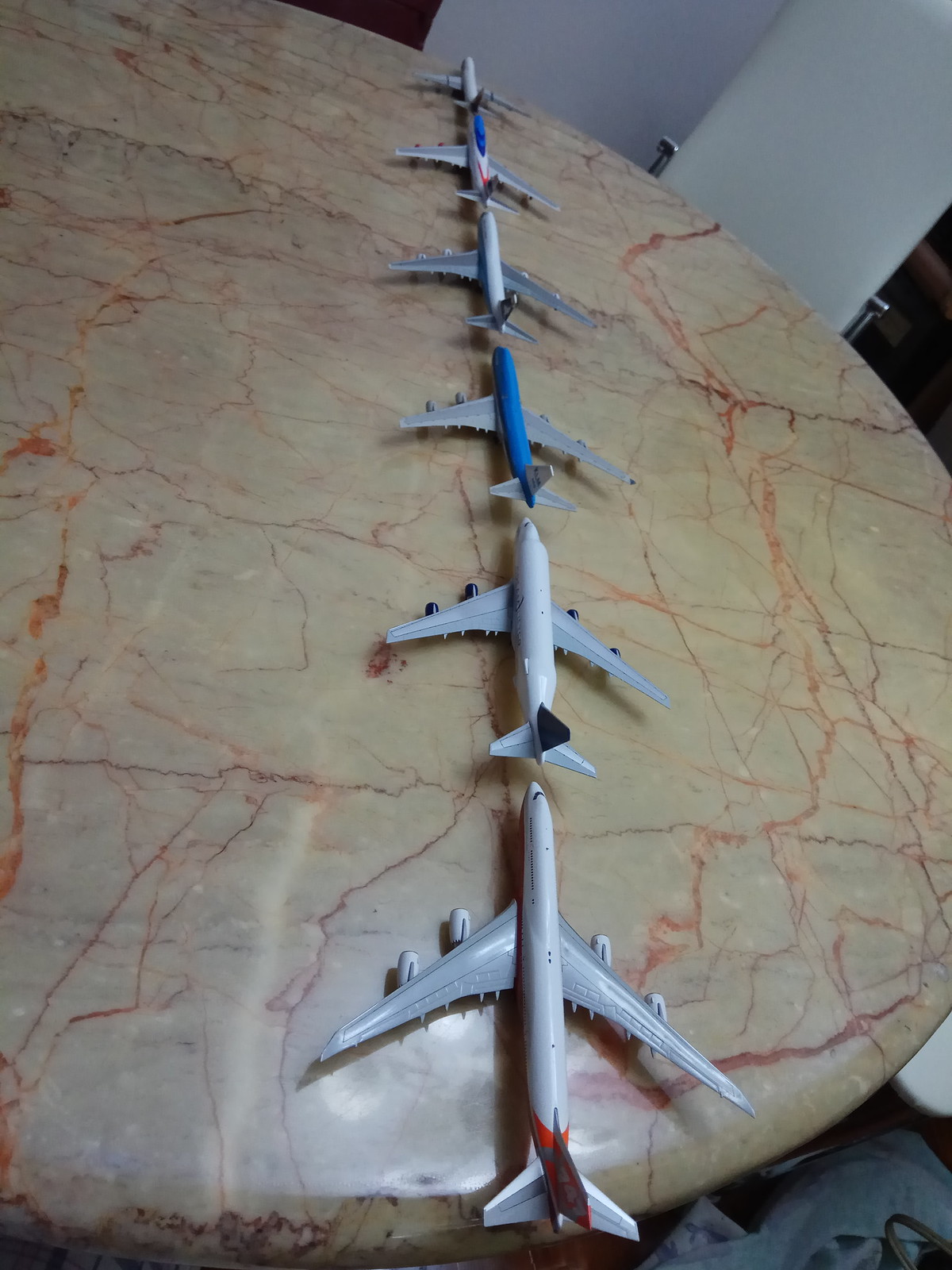The photograph captures six model airplanes meticulously arranged in a vertical line on a round, marbled tabletop. The tabletop, with its creamy beige color interspersed with striking red and brown marbling patterns, adds a luxurious backdrop to the scene. The table's reflective surface highlights the carefully placed airplanes, enhancing their vibrant details.

Starting from the bottom, the first model airplane is gray with distinctive orange markings near the tail, followed by a white airplane with a black rudder on its tail. Above it, a blue aircraft with silver wings creates a standout visual contrast. The next one up is predominantly white, featuring silvery wings. A gray airplane with blue and red stripes on its tail follows. Finally, the topmost airplane is a clean slate gray, contributing to the cohesive yet varied display. All the airplanes feature sleek, commercial jet-like designs with wings extending toward the back in a V-shape, creating an impression of streamlined motion as they touch end-to-end ascending through the image.